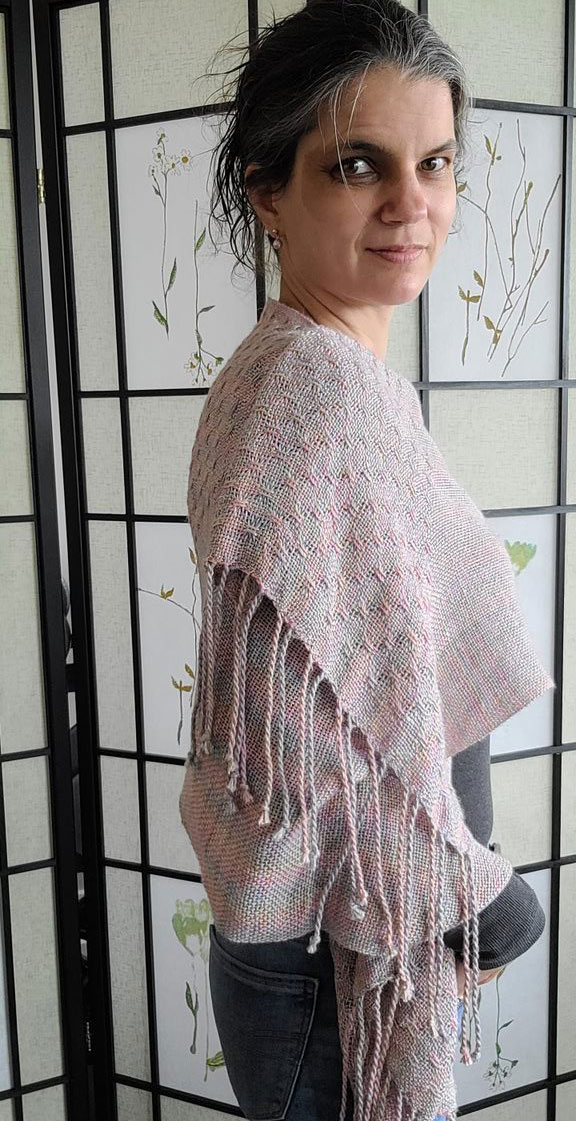This photograph captures an enigmatic middle-aged woman standing indoors in front of a decorative privacy divider with a floral design. Her dark auburn hair, streaked with gray, is pulled back into a messy bun with strands sticking out, amplifying the casual nature of her appearance. She sports dark eye makeup, visible bags, and shadows under her eyes, which contribute to her somewhat tired yet defiant expression. Her attire includes a pastel-colored, light pink and gray hand-woven shawl with long fringe, draped over a gray shirt and charcoal-colored jeans. She accessorizes with pearl earrings. The woman is positioned sideways, turning her head to the right to gaze into the camera with a complex mix of aloofness and a slight smile, giving her an ambivalent, almost mysterious demeanor.